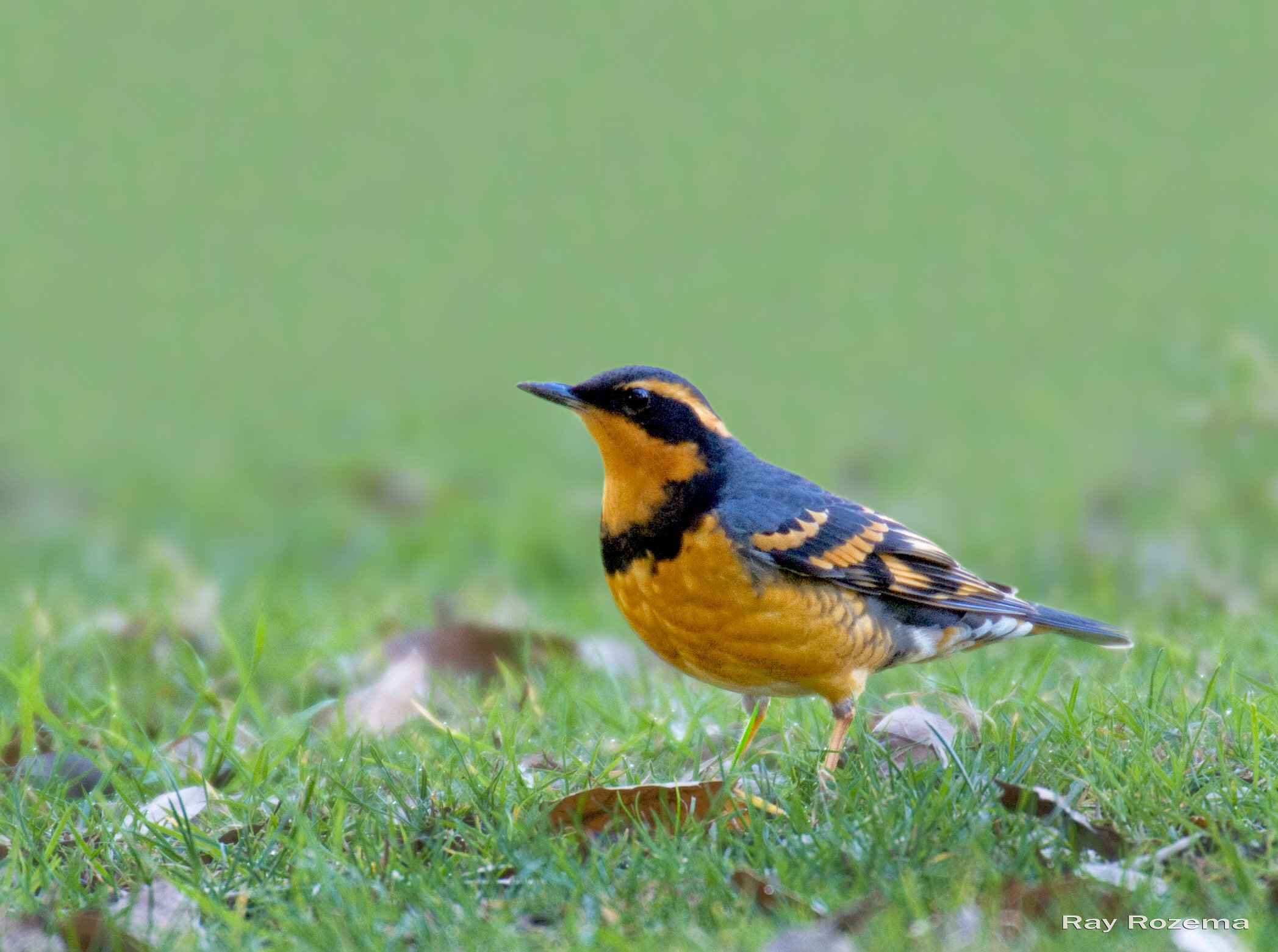The photograph features a small bird standing in green grass, surrounded by scattered brown leaves. The bird, positioned centrally towards the right and facing slightly upwards to the left, captures attention with its striking yellow belly and a head that shares the same yellow hue. Distinguishing features include black stripes running through its head and a black beak. The bird’s wings are a dark blue-black color, and it sports a black line around the throat area. Towards the tail, its plumage lightens to a shade of lighter gray. Notable are its yellow legs and talons. The background of the image is predominantly out of focus, maintaining a green hue consistent with the grassy setting. "Ray Rosema" is visibly inscribed in white letters at the bottom-right corner of the photo.